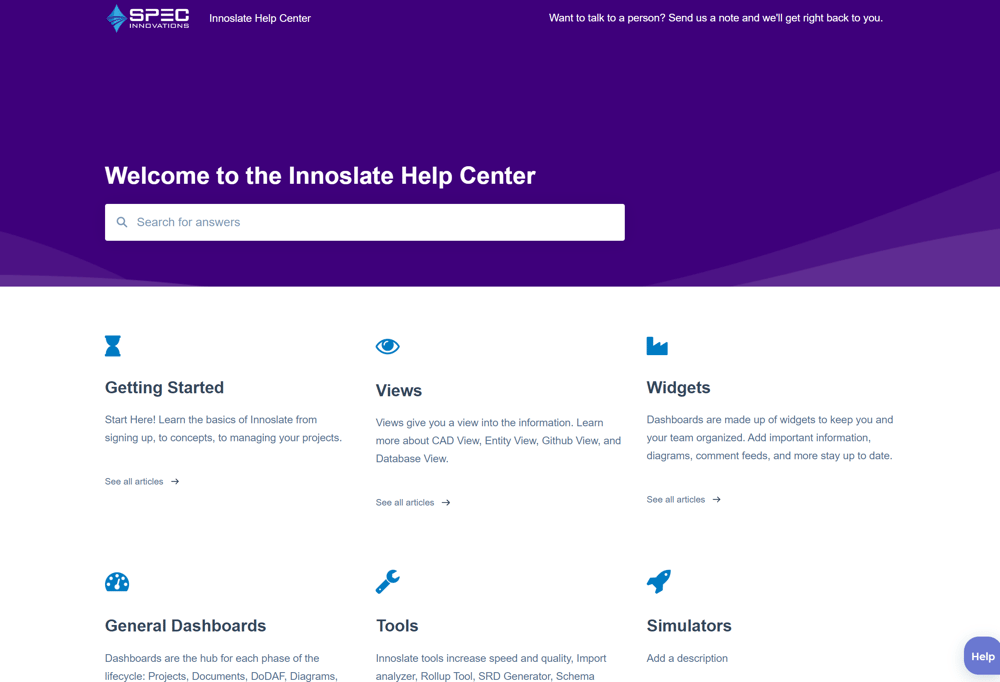This is a screenshot from the Speck Innovations website. On the left side, the company's logo is prominently displayed, depicting a blue diamond. To its right, in a distinctive uppercase font, is "S-P-E-C," with the word "Innovations" in small white text below it. Adjacent to the logo, the header text reads "Insulate Help Center." Further to the right, in small white text, a message states: "Want to talk to a person? Send us a note and we'll get right back to you."

Below this header, the background transitions to a purple hue, atop which sits a search bar. Above the search bar, large white text welcomes users with the phrase: "Welcome to InnoSlate Help Center." Below this heading are six distinct options for users to explore: "Getting Started," "Views," "Widgets," "General Dashboards," "Tools," and "Simulators." At the very bottom right corner of the screenshot, there's a small blue button featuring a help icon, ready to assist users with their inquiries.